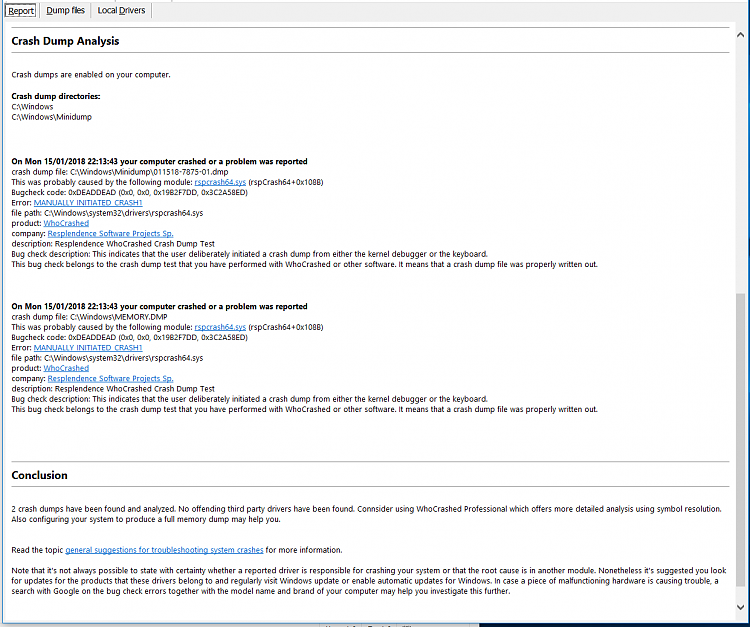**Screenshot of Crash Dump Analysis Report**

The screenshot displays a detailed crash dump analysis report on a computer screen.

- **Top Section:**
  - Three small boxes with black labels are located at the top, titled "Report," "Dump Files," and "Local Drives."
  - The interface has a light gray border across the top and down the side. On the right, a dark gray slider is visible, with an up arrow and a down arrow at the bottom.

- **Main Header:**
  - Between two gray lines, in bold black letters, the title "Crash Dump Analysis" is displayed.
  - Below the title, the text "Crash dumps are enabled on your computer" is mentioned.
  
- **Crash Dump Directories:**
  - "Crash dump directories" is bolded, followed by paths: 
    - `C:\Windows`
    - `C:\Windows\Minidump`
    
- **Crash Reports:**
  - **First Report:**
    - Date and Time: "On Wednesday, 15/01/2018 at 22:13:43"
    - Incident: "Your computer crashed or a problem was reported."
    - Crash file provided.
    - Potential Cause: "This was probably caused by the following module that is outlined in blue: Error manually initiated crash."
    - Product and Company: "The product [WhoCrashed] by Resplendent Software Projects."
    - Description: "It was a crash dump test."
  - **Second Report:**
    - Date and Time: "On Monday, 15/01/2018 at 22:13:43"
    - Incident: "Your computer crashed or a problem was reported."
    - Same crash file provided.

- **Conclusion Section (In bold between two gray lines):**
  - "Two crash dumps have been found and analyzed. No offending third-party drivers have been found."
  - Recommendation: "Consider using WhoCrashed Professional, which offers more detailed analysis using symbol resolution."
  - Additional Advice: "Configuring your system to produce a full memory dump may help you."
  - A suggested reading link in blue: "General suggestions for troubleshooting system crashes for more information."

- **Additional Notes:**
  - "Note: It is not always possible to state with certainty whether a reported driver is responsible for crashing your system or that the root cause is another module."
  - Recommendations:
    - Look for updates for the projects that these drivers belong to.
    - Regularly visit Windows Update or enable automatic updates for Windows.
    - If malfunctioning hardware is suspected, a search using Google with the bug check errors, model name, and brand of the computer may help further investigate.

This detailed screenshot is an example of how critical system information and errors are reported in crash dump analysis, aiding in troubleshooting and resolving system crashes.